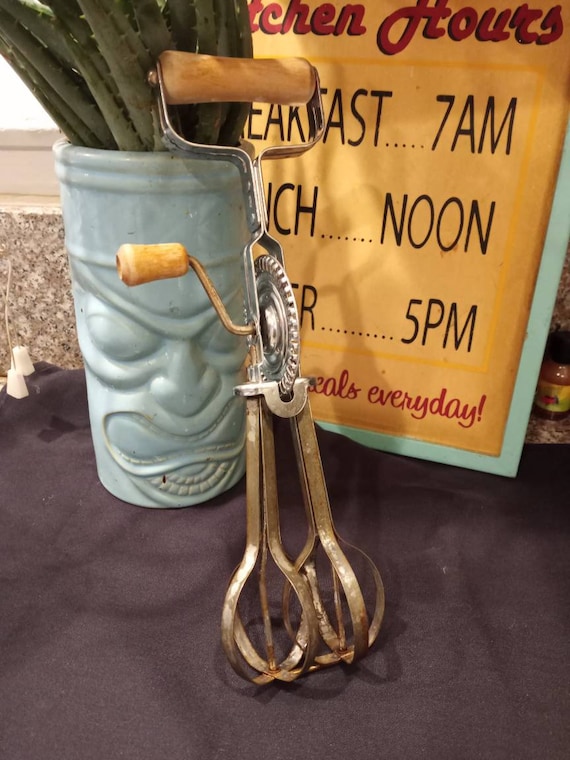The photo showcases a vintage kitchen scene centered around a hand-powered beater with a wooden handle and a small lever on the side that spins two metal whisks at the bottom. Positioned in the middle, the beater hints at its use for whipping eggs or batter. Behind it to the right, there's a vintage-style menu board with red and black lettering reading "Kitchen Hours," specifying breakfast at 7 a.m., lunch at noon, and dinner at 5 p.m., though some text is cut off, it mentions "meals every day." This sign is on a mustard-yellow paper framed in a light turquoise border. To the left, there is a blue ceramic planter designed to resemble a tiki face, with a plant resembling aloe sprouting from it. The scene is set on a black cloth, likely on a counter, with a glimpse of tiles and a window sill in the background. A small jar is partially visible behind the menu board.